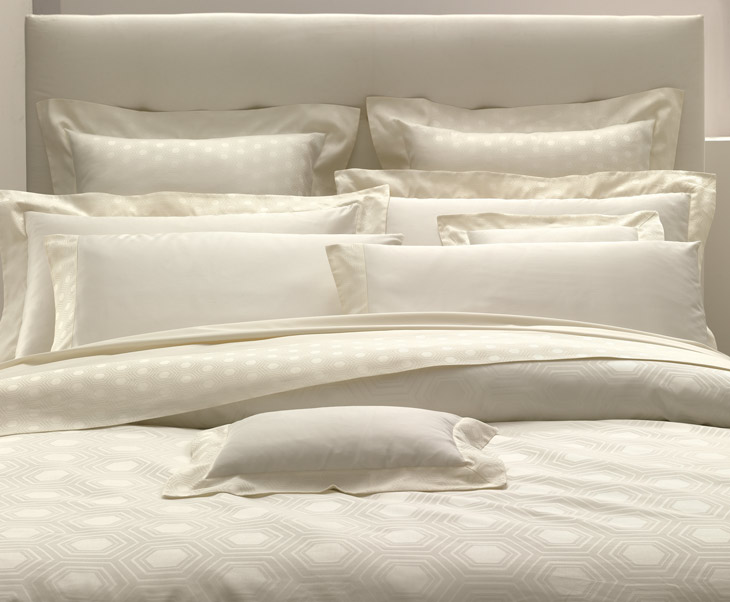This image depicts a lavish, cream-colored bedroom setup centered around a double bed. The bed has a striking headboard upholstered in a fabric that blends seamlessly with the creamy off-white walls. There are nine satin pillowcases visible, their lustrous finish adding a touch of luxury. Seven of these pillows are stacked against the headboard, creating a plush backdrop. A smaller, satin-cased pillow sits prominently in the center. The bedding features elegant sheets with a subtle hexagonal pattern, hinting at a high thread count and an expensive taste. The comforter, also made from shiny satin material, is somewhat unusually folded up in front of the pillows, rather than laid out beneath them. The overall color scheme of various shades of ivory and the sheen of the materials throughout emphasize an impression of decadence and sophistication.